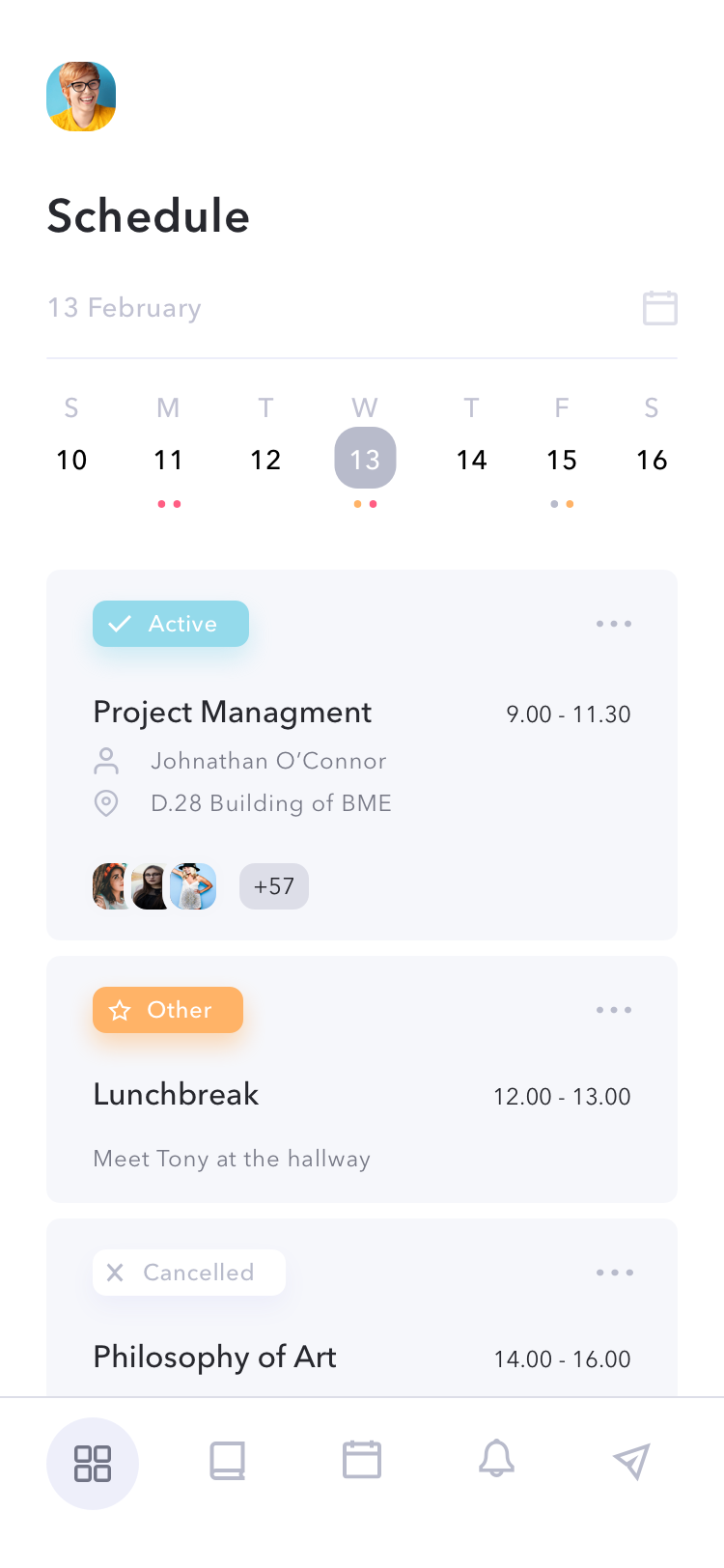The screenshot displays a scheduling app, with the header labeled "Schedule". The profile picture on display belongs to a person who appears somewhat androgynous, likely female, with a nerdy appearance characterized by glasses and short-ish hair. She is wearing a mustard yellow t-shirt and has a fair complexion, and she is smiling.

The schedule is in a week view format, spanning from Sunday, February 10th, to Saturday, February 16th, with the current focus on Wednesday, the 13th. The detailed events for that day are listed as follows:

1. **Project Management Meeting**
   - **Time:** 9:00 AM - 11:30 AM
   - **Participants:** Jonathan O'Connor and several others, identifiable by their profile pictures.
   
2. **Lunch Break**
   - **Time:** 12:00 PM - 1:00 PM

3. **Philosophy of Art Class**
   - **Time:** 2:00 PM - 4:00 PM

The context of these events remains uncertain; it could pertain to a work-related schedule or an academic one, suggesting a busy day with back-to-back commitments. If it is work-related, it indicates a full-time job, raising questions about how she manages such a packed schedule.